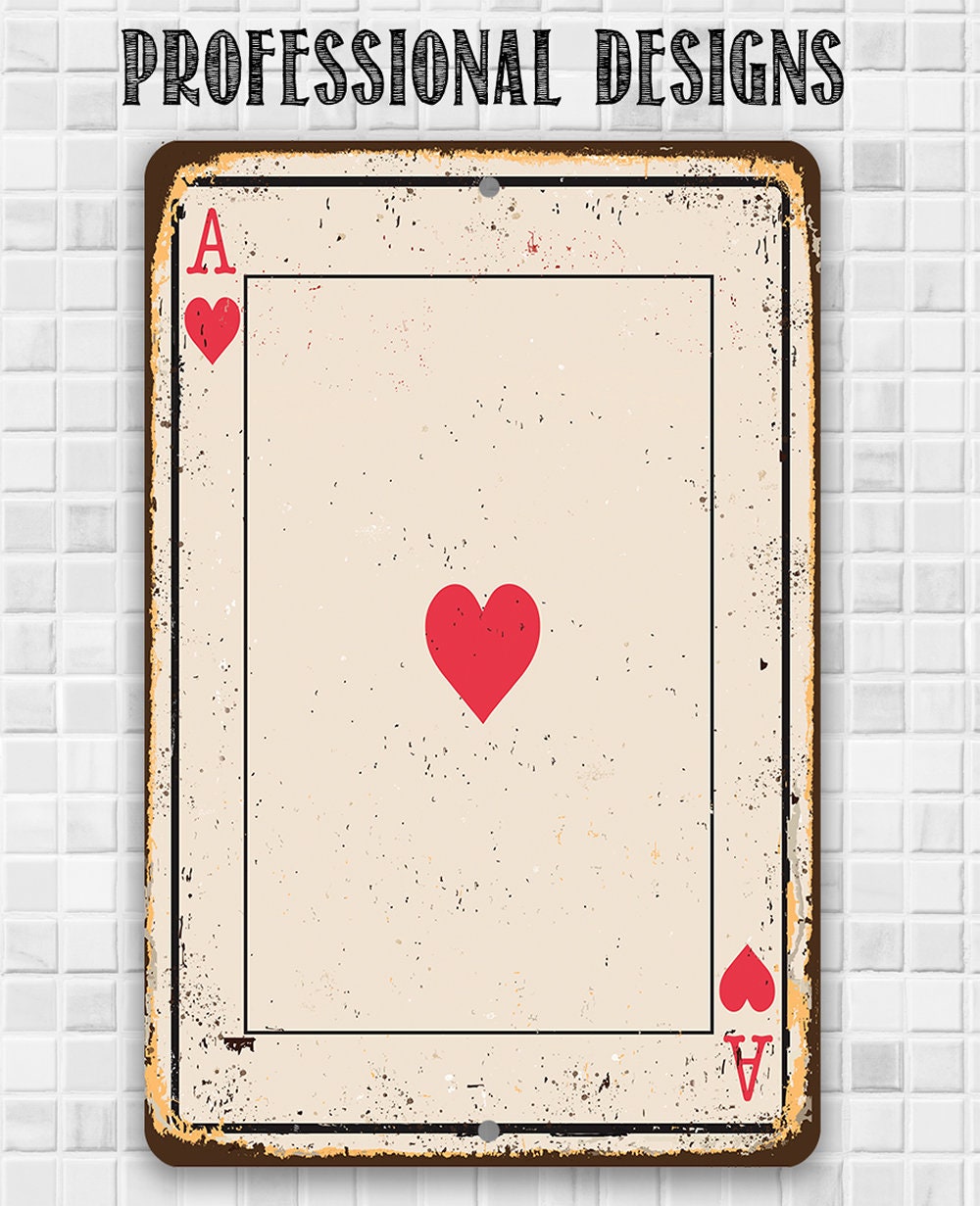The image features an advertisement with a vertical rectangular orientation. The background is a light gray tiled wall composed of uniformly small squares arranged in horizontal rows. In the center, there's a prominent metallic Ace of Hearts playing card, characterized by its rusted and damaged edges, indicating its metal construction. The card showcases a red letter "A" accompanied by a red heart symbol in both the top left and bottom right corners, as well as an additional large red heart in the center. Black flecks and dust are scattered across the card's surface, adding to its weathered appearance. Above the card, in large, bold black capital letters, the text "PROFESSIONAL DESIGNS" is displayed, emphasizing the nature of the advertisement – likely promoting a professional design company's work. The colors on the card include white, black, yellow, brown, and shades of gray, enhancing the contrast against the tiled backdrop.